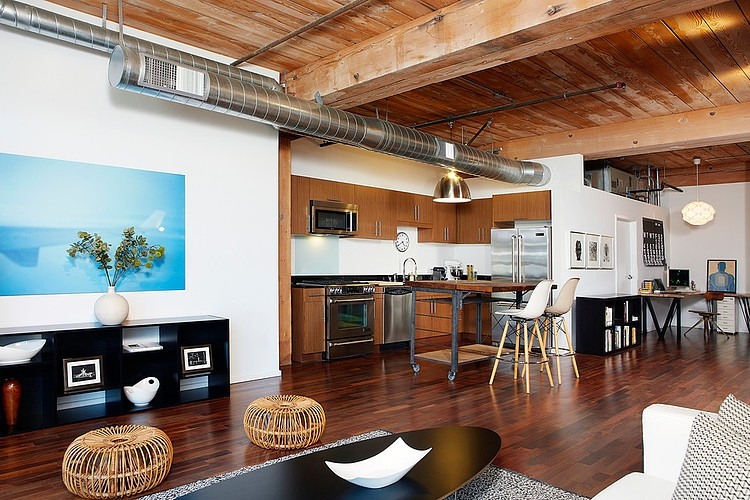The image showcases an upscale loft with an open layout that seamlessly combines a living area and a kitchen. The space is accentuated by beautiful, shiny reddish-brown wood flooring and light-colored wooden ceiling paneling with rafters. The walls are predominantly white, giving the space a bright and airy feel.

In the living area, a light-colored couch adorned with checkered black and white pillows faces a black coffee table that features a white centerpiece. A plush rug lies beneath this setup, anchoring the seating area. Against the left wall, there is a projector screen above a black, hollowed-out storage unit, which houses a variety of home decor items, including pictures and books. On top of this unit sits a white vase with two green leaves beside a plant. Two round wooden baskets complement the decor in front of the storage unit.

The kitchen, visible towards the back of the image, boasts top and lower cupboards in the same light wood tone as the ceiling. A large silver refrigerator, a rolling island, and modern appliances including a microwave and dishwasher highlight the kitchen's functionality and style. A small office area with a computer and additional shelving is tucked to the right, offering a perfect blend of work and leisure in this inviting, open-concept loft.